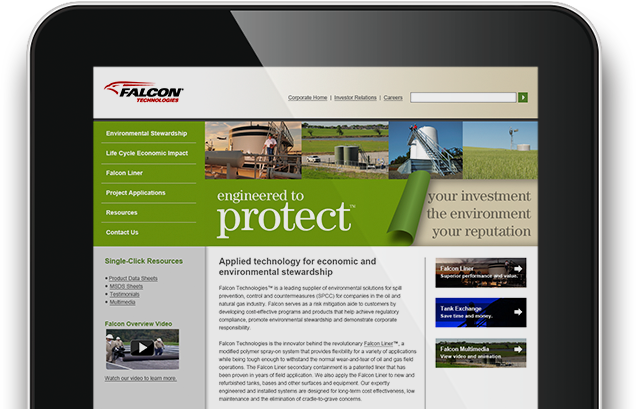The image captures a tablet with a sleek, black border, slightly illuminated by natural light creating a gradient from jet black on the left side to light gray on the right side. The tablet screen displays the website of Falcon Technologies. At the top of the webpage, there is a tan-colored header featuring the company’s logo: a red bird facing left, the word "Falcon" in black, and "Technologies" in red underneath. Beneath the header, navigation tabs labeled "Corporate Home," "Investor Relations," and "Careers" are visible alongside a white search box with a green submit button.

Prominently, a green banner stretches across the page. On the left side of the banner is a menu with gray lettering that lists options including "Environmental Stewardship," "Lifecycle," "Economic Impact," "Falcon Liner," "Project Applications," "Resources," and "Contact Us." Adjacent to the menu, the banner features four images showcasing various storage silos.

Below the banner, centered text reads "Engineered to Protect" in white on a green background that visually resembles a rolled-out grass mat. To the right, a tan-colored section with black lettering states, "Your Investment, The Environment, Your Reputation."

In the lower portion, the left section highlights "Single Click Resources" in green, accompanied by various menu options and a link to a Falcon overview video. The middle section presents a detailed text block about "Applied Technology for Economic and Environmental Stewardship." To the right, three vertically arranged boxes provide information on "Falcon Liner," "Tank Exchange," and "Falcon Multimedia."